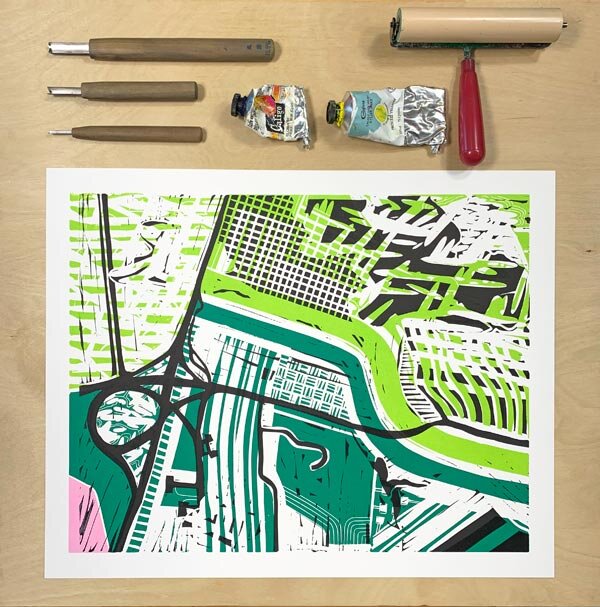This detailed photograph showcases an artist's workbench featuring a variety of tools and an incomplete piece of art. The tabletop is made of light tan wood, setting a neutral backdrop for the vibrant activity. At the top of the image, there are three tools with metal tips and dark brown wooden handles, likely used for scraping or carving. Positioned next to these are two nearly depleted tubes of paint with silver bases and labels, one of which has a teal color on top. Adjacent to the paint tubes lies a red-handled paint roller with a tan-colored roller.

Dominating the lower part of the photograph is the artist's canvas, a compelling work that resembles an aerial map. The artwork is detailed with a mix of colors, including various shades of green, vivid lime green, and accents of pink and black. The elaborate design features intricate lines depicting roads, interchanges, fields, and possibly the tops of buildings, with a white background enhancing the vibrancy of the colors. The composition of tools and art provides a snapshot into the meticulous and colorful process of the artist at work.